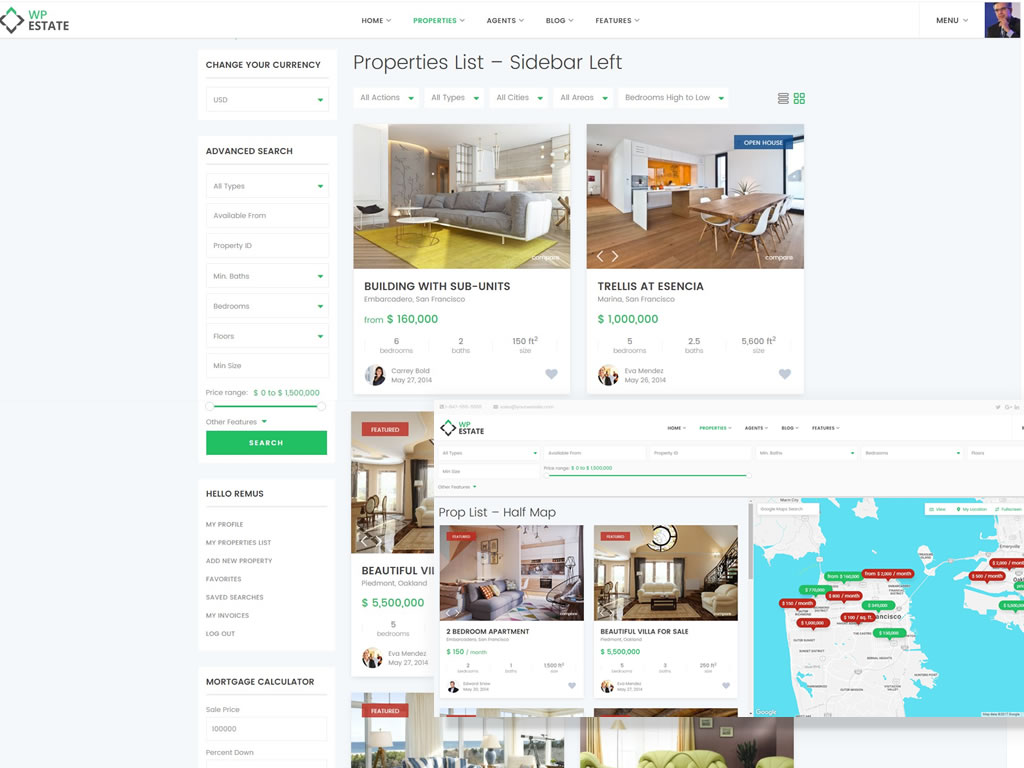Screenshot Description:

The screenshot captures a website interface for WP Estate, identifiable by the distinctive logo in the upper left-hand corner where "WP" is displayed in green and "Estate" in black. Central to the image are property listings, introduced by the header "Properties List, Sidebar Left." 

Prominently featured is a property priced at $160,000, described as "buildings with subunits." Adjacent to this listing is another property titled "Trellis at Essentia." Beneath these listings, a map view displays locations of properties, each marked with corresponding pins.

On the upper right-hand side, there is a profile picture accompanied by a menu drop-down selection. The left-hand sidebar offers an array of search filters, allowing users to refine their property search by currency, property types, accommodation, property ID, minimum bathrooms, bedrooms, floors, size, and a price scale, culminating in a search button.

Additionally, the sidebar presents menu options including "Profile," "My Profile," "Property List," "Favorites," and "Logout," along with a few others that are not fully legible. A built-in mortgage calculator is also available for users' convenience.

The entire interface is set against a light gray background, providing a clean and user-friendly navigational experience.